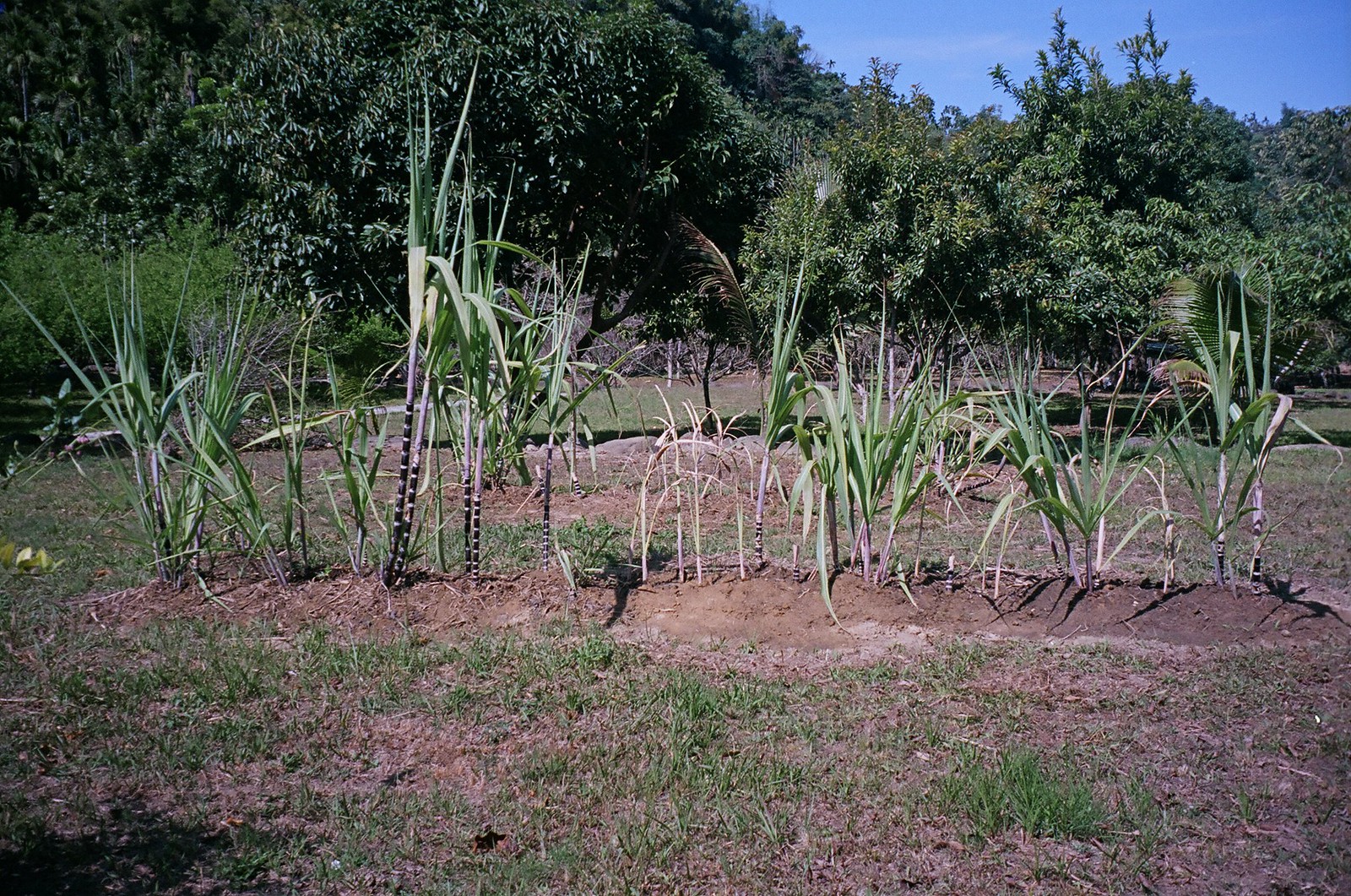In this vibrant outdoor photograph taken in bright sunlight, we see a small garden or farm against the backdrop of lush, overgrown bushes and diverse trees, with a glimpse of the blue sky in the top right corner. The red-tinted ground features patches of grass interspersed with bare dirt. Prominently emerging from a central section of oblong dark blue and dark brown soil are several tall, spindly plants bearing a variety of broad, green, palm-shaped leaves that glisten in the sunlight. Some of these plants have a distinct black and white striation at the base of their stems, adding a unique texture contrast. While the central plants vary slightly in appearance, suggesting they might be related species or at different growth stages, the overall scene is one of verdant, organic beauty. The thick blades of leaves and grass in the foreground complement the robust greenery of the trees in the background, creating a serene and flourishing garden vista.